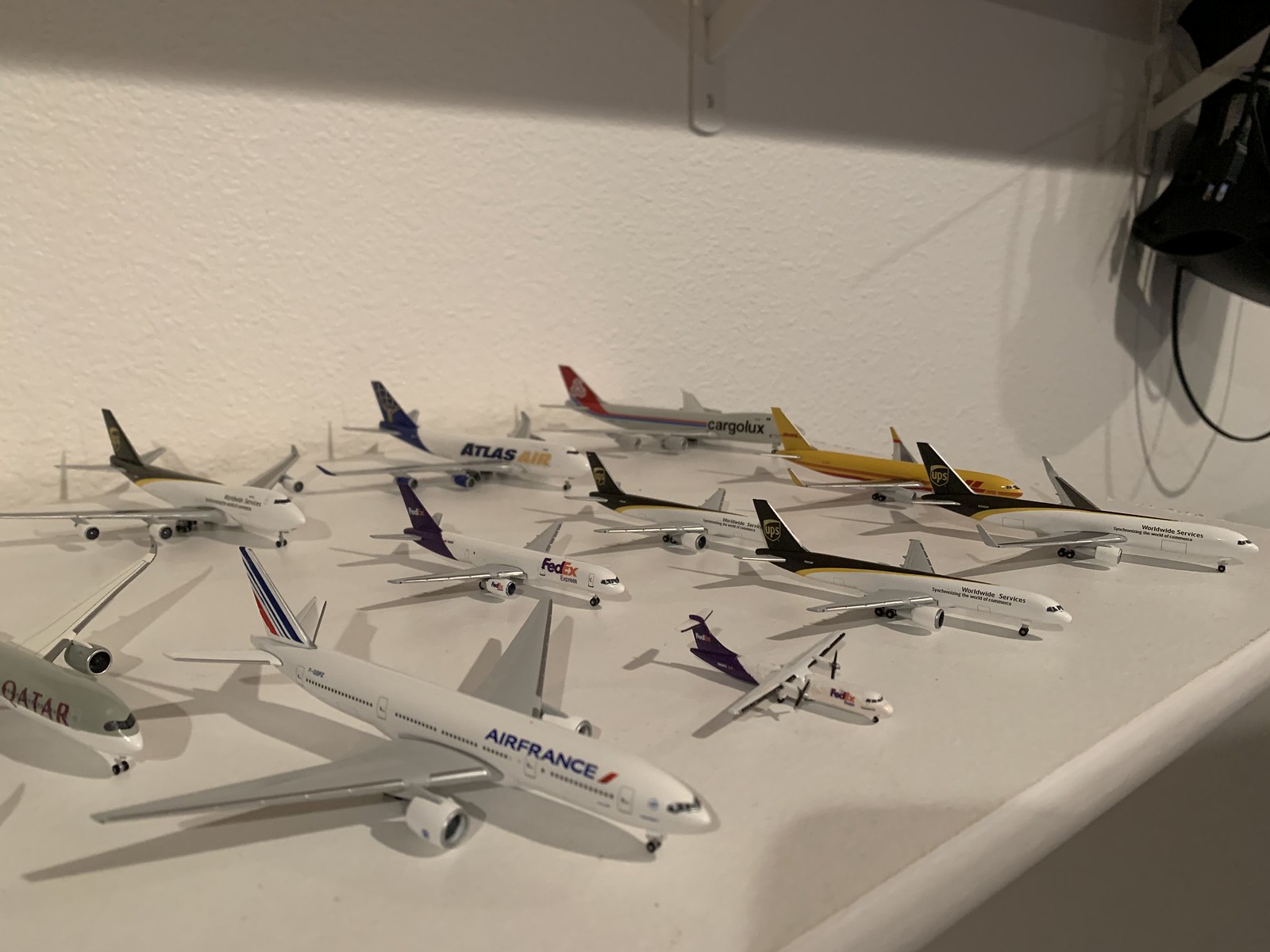The indoor color photograph showcases a meticulously arranged white shelf against a slightly textured white wall, revealing 15 to 16 miniature model airplanes in a three-quarter profile, all oriented with their noses pointing to the right. The collection includes airliners such as a front-left Qatar Airways model, an Air France plane with a red-striped logo and a tricolor back wing, and a DHL plane in yellow with a large, partially obscured "L." Towards the back, we see models of FedEx and Atlas Air planes, along with a Cargolux model featuring a red and white back wing. Additionally, two more planes bear the UPS logo on their tails. The light source from the right casts slight shadows to the left of the models, enhancing the detailed exteriors that mimic their real-life counterparts.